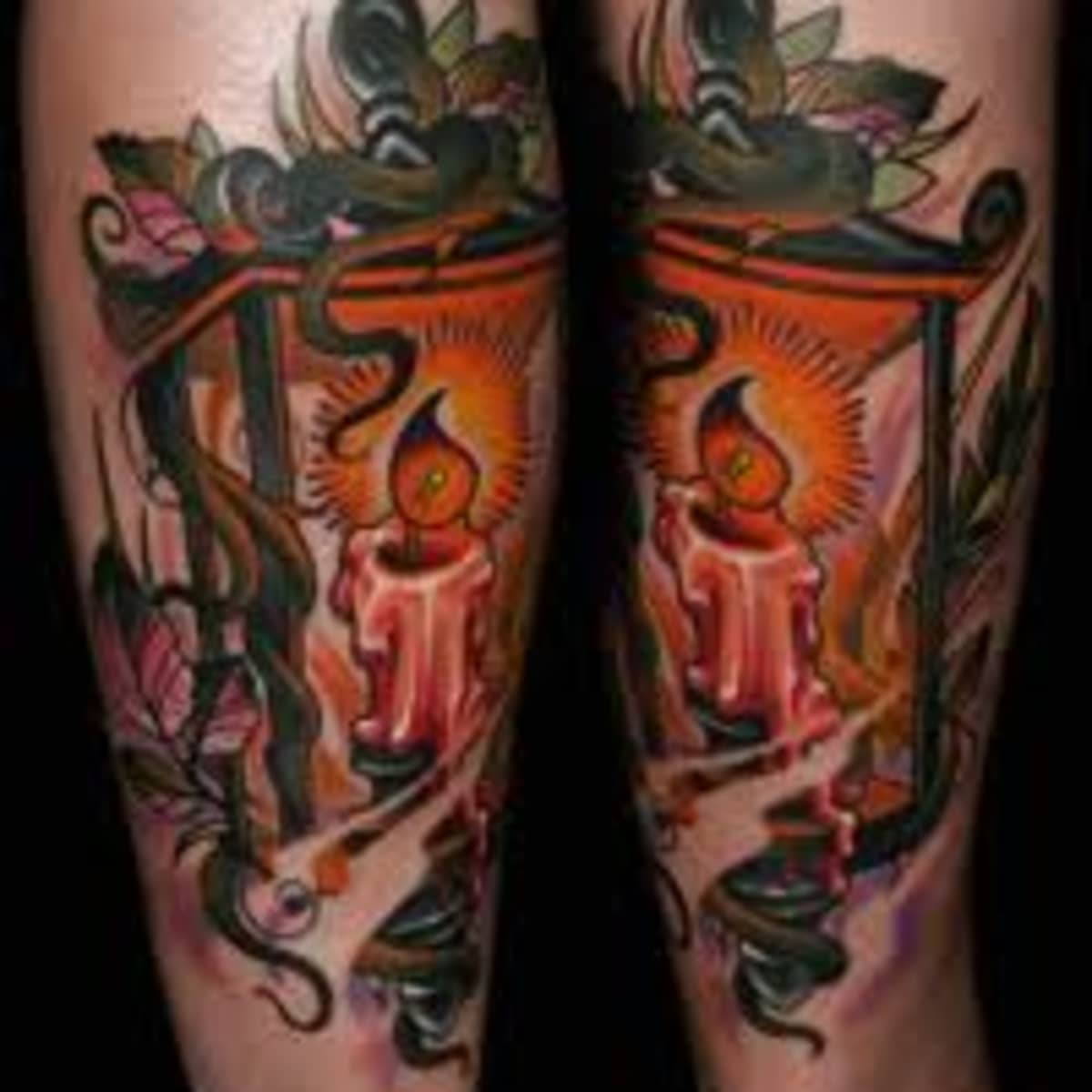The image showcases a close-up of two pale limbs, either arms or legs, adorned with matching tattoos. Each limb features a vividly detailed, pink candle at the center, glowing with an orange flame and accompanied by melting wax. The candles are encased in ornate, green lantern-like structures, which are adorned with intricate vines and leaves that exhibit varying hues of green, sprinkled with touches of pink and pinkish-purple. These elaborate tattoos cover an extensive area, possibly extending from the upper thigh down to the ankle or from the upper arm to the wrist. The background of the image is completely black, accentuating the intricate design and vibrant colors of the tattoos.